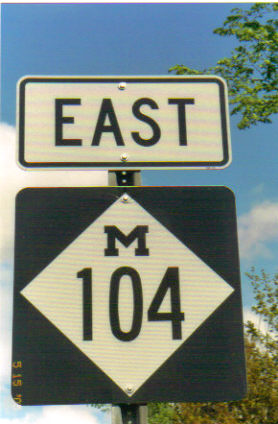The image depicts a close-up of a road sign mounted on a metal pole with small circles. The top sign is a white rectangle with a black border and reads "EAST" in black lettering. Directly below it, attached by two silver screws, is a square sign with a black background featuring a white diamond in the center. Inside the diamond, "M104" is displayed with the "M" in black lettering at the top and "104" in larger black numbers beneath it. Both signs have rounded corners and are set against a background of trees in varying stages of fall foliage, indicating the season is either spring or summer. The sky behind the sign is a vibrant blue, dotted with puffy white clouds on the left and a few wispy ones to the right of the square sign. Additionally, there is a partially visible yellow timestamp in the lower left corner that reads "51500" or possibly "2000". There's nothing else of significance in the image, and the perspective of the photo suggests that the viewer is looking up at the sign.